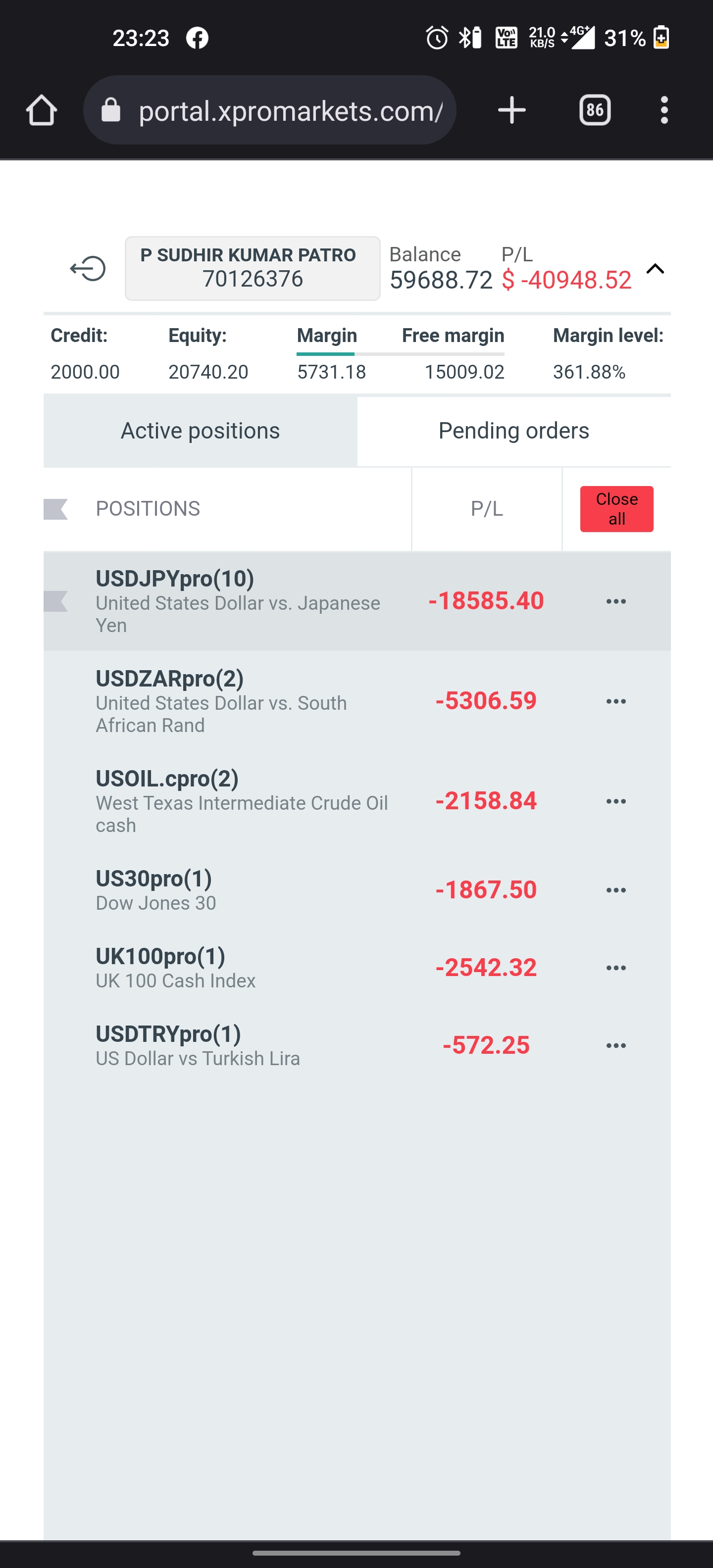This image is a screenshot from a smartphone displaying a website. The website URL visible at the top reads "portal.xpromarkets.com" in white lettering against a black background banner. Positioned below the banner, the website features a clean, white background with black text detailing account information. The information includes various types of currencies and their respective amounts within the account, suggesting that this is a platform related to banking or investment management. The interface appears to be user-friendly and straightforward, allowing users to easily view and manage their financial assets.